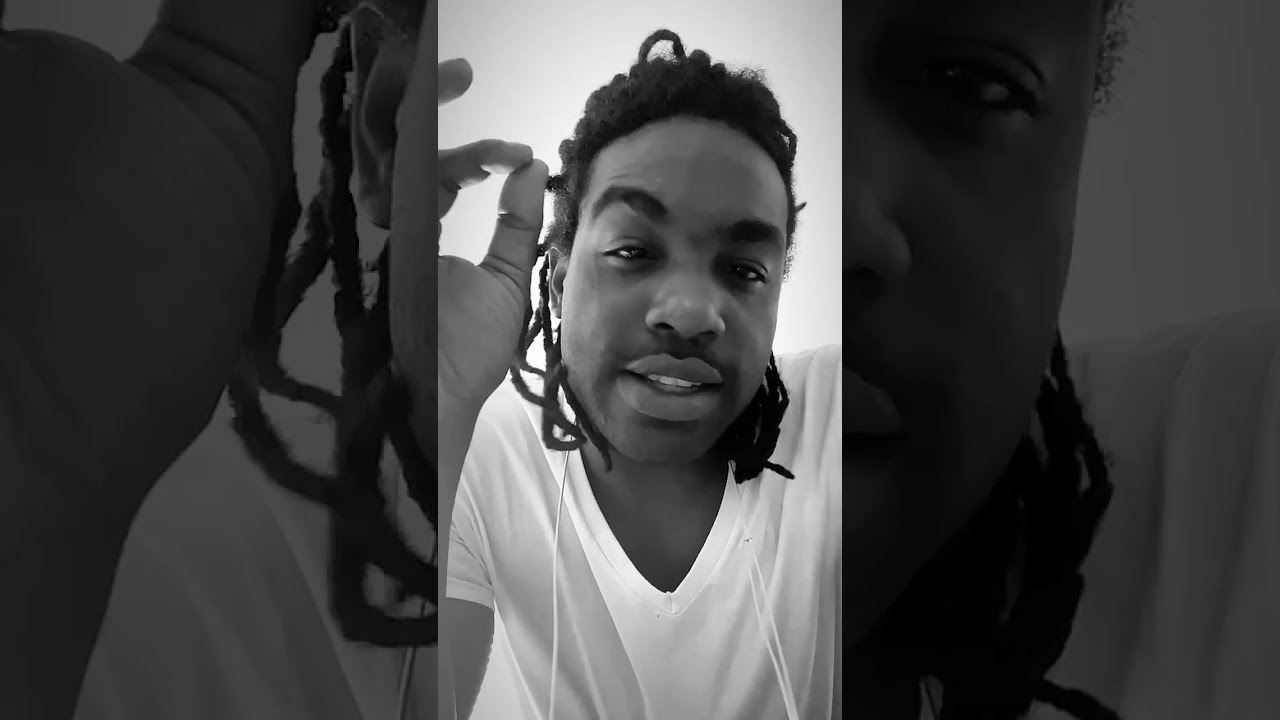The image is a clear, centered digital photograph of a dark-skinned man with braided hair falling down to his neck behind his ears. He has dark eyebrows and a light mustache, with his mouth slightly open, showing a few teeth below his upper lip, suggesting he is speaking. He is wearing a white, v-neck, short-sleeved t-shirt, and white earbud wires are visible around his neck. His right hand is partially visible on the left side of the image, with thumb and index finger touching each other, though it's partly cut off. The background features close-up gray versions of the same image, creating a mirrored effect on either side. The man looks directly at the camera, possibly engaged in a live video session, as he appears to be speaking calmly.